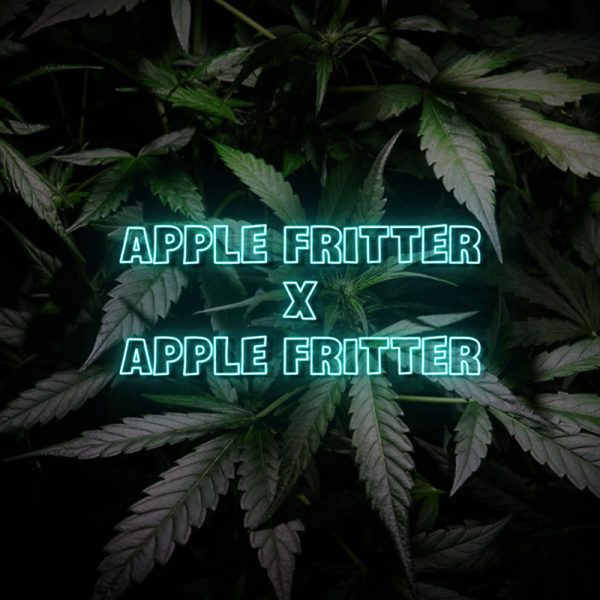In the dark, dimly lit image, a collection of large, healthy marijuana leaves forms a dense pile in the center, their green hues appearing lighter at the ends. The leaves are sharply pointed and lack any visible buds. The background fades into near-blackness at the corners, creating a moody ambiance. Overlaid in the center of the image is text that glows with a blue neon appearance. The top and bottom rows of the text spell out "APPLE FRITTER" in capitalized letters, while the middle row features a single, centered "X." This text appears to shine, as if illuminated, standing out starkly against the dark backdrop.